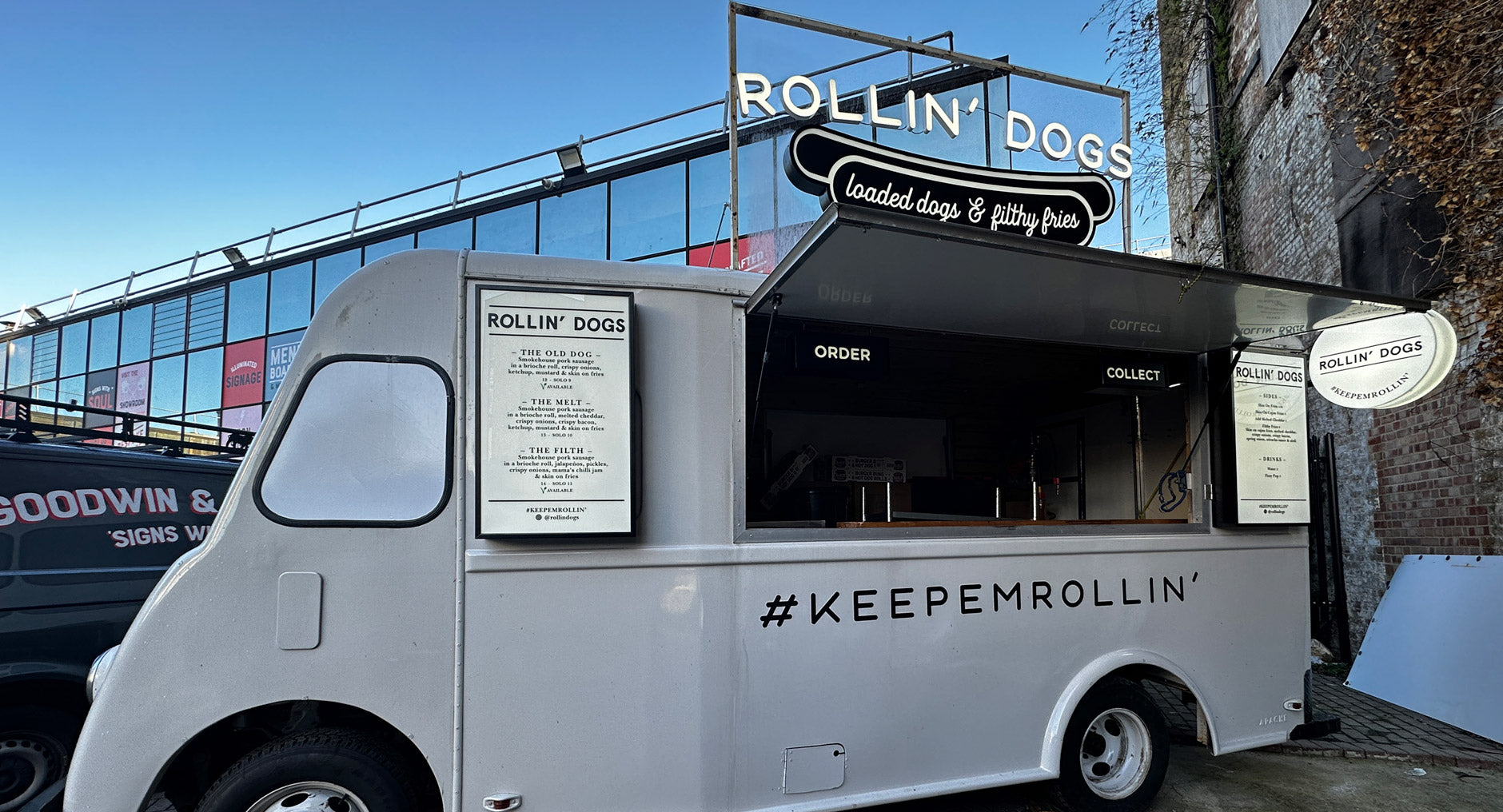This image showcases a beige concrete-colored food truck named "Rolling Dogs" prominently positioned in the center. The truck's windshield appears painted in, suggesting it may be stationary rather than mobile. The truck features dual menus on either side of a service window, from which customers order their meals. Above the service area, the text "Rolling Dogs" is clearly visible, along with additional signage for "Loaded Dogs" and "Philly's Pies." Below the serving area, there's a hashtag phrase, "Keep Keepin Rolling." The scene also includes a second vehicle situated to the left of the food truck, a fence partially enclosing the area, and the side of a brick building adorned with multiple signs. The dominant colors in the photograph are grays, reds, dark blues, sky blue, a yellowish, dead leaf color, and black, contributing to the overall urban and eclectic atmosphere.